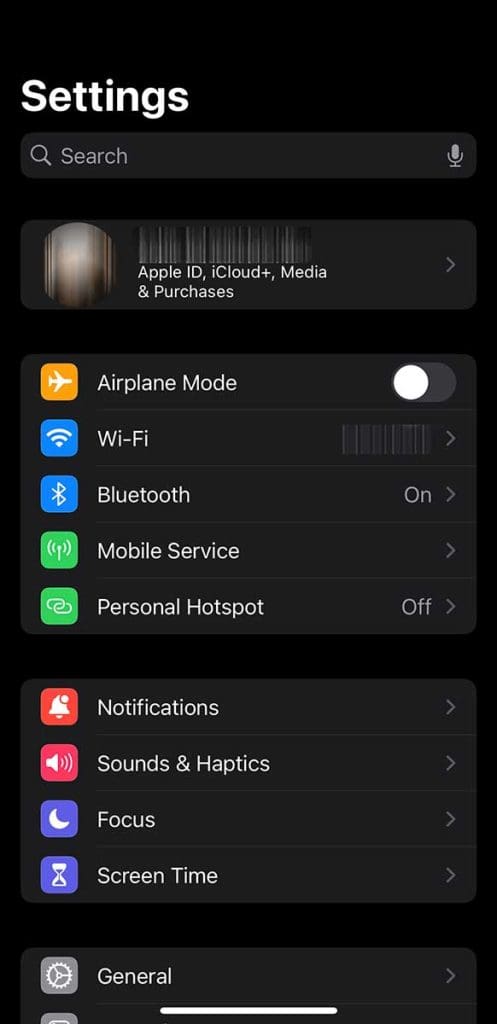The image features a black background with the word "sentence" prominently displayed at the top in large white letters. Beneath this, there is a search bar with icons for a magnifying glass and a microphone on the right side. Below the search bar, a box contains a blurred-out picture and blurred text, with the words "Apple ID, iCloud Plus, Media and Purchases" clearly visible underneath.

Further down, two sections are displayed. The left side of each section shows icons representing various functions, while the right side has corresponding on/off switches. The top section lists "Airplane Mode" (turned off), "Wi-Fi," "Bluetooth" (turned on), "Mobile Service," and "Personal Hotspot" (turned off). The bottom section includes labels for "Notifications," "Sound and Haptics," "Focus," "Screen Time," and "General."